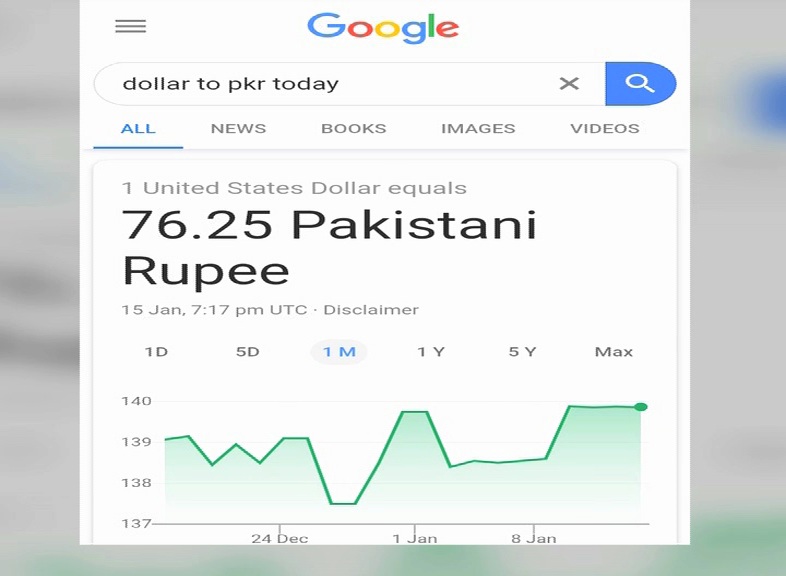The image is a horizontally stretched screenshot from a mobile device, capturing a partial view of the user's phone screen while using Google. The Google logo is prominently displayed at the top of the screenshot. On the upper left side, a hamburger navigation icon is visible. The person has searched for the term "dollar to PKR today." The search results page is shown in the "All" category, which includes options to view news, books, images, and videos.

Central to the image is a graph depicting the exchange rate of one United States dollar (USD) to Pakistani rupees (PKR). According to the snapshot, one USD equals 76.25 PKR as of January 15th, 7:17 PM UTC. Below this conversion rate, there is a link to a disclaimer. The graph illustrates the fluctuation of the Pakistani rupee's value over a selected time frame, with options to view data for one day, five days, one month, one year, five years, or the maximum available period. The selected time frame is one month, covering the range from December through January.